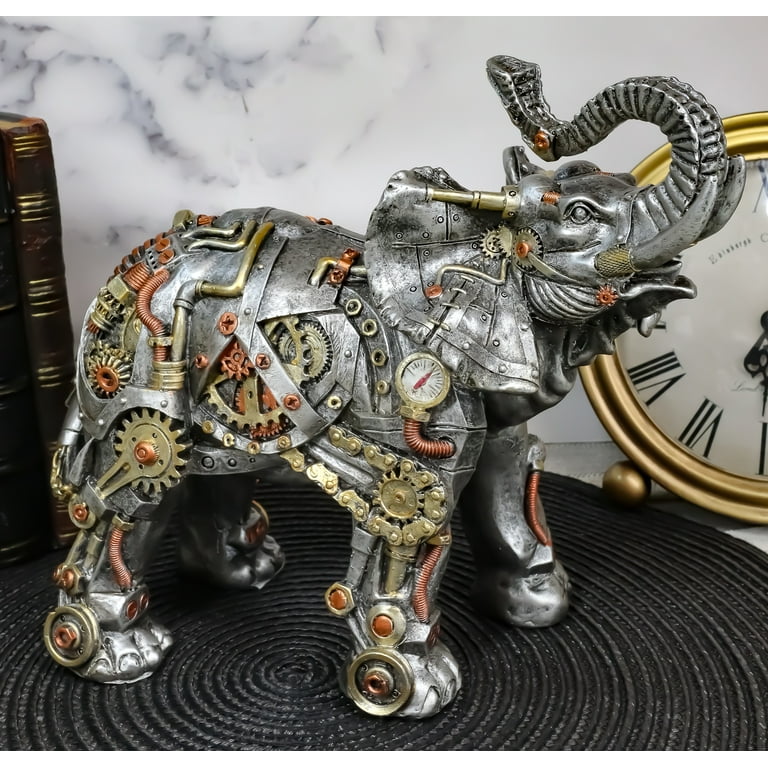This photograph features an intricately detailed statue of an elephant, masterfully crafted to embody a steampunk aesthetic. Constructed from burnished pewter, the elephant sculpture incorporates a range of metallic elements, including gold and bronze cogwheels, chains, screws, and even bicycle chain links, giving it a mechanical, robot-like appearance. The elephant is adorned with a multitude of features, such as a lifted trunk, prominent tusks, visible tongue, and well-defined ears, all of which accentuate its lifelike semblance despite its mechanical components.

The statue is placed on a round, black woven placemat set atop a flat, gray surface, likely a desk or table. Enhancing the scene, a large analog desk clock with a white face, black Roman numerals, and a gold frame sits to the right of the sculpture. The background reveals a marble-patterned wall in white and gray tones, providing a contrasting backdrop to the artwork. To the left of the elephant, a book stands upright, its spine visible, adding an intellectual charm to the setting. This decorative piece effectively combines elements of steampunk art with everyday objects, creating a unique and fascinating desk ornament.